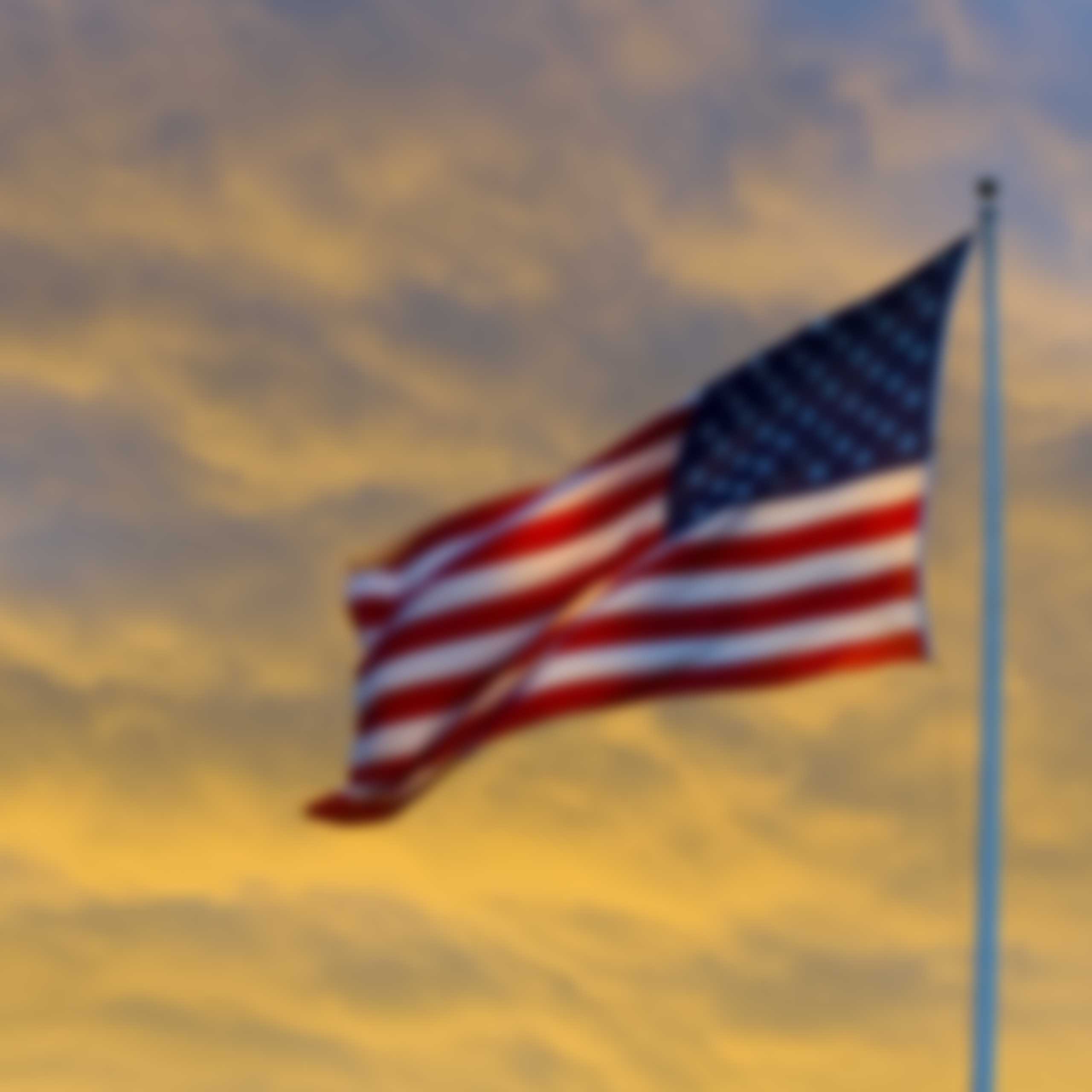This is a photograph of an American flag waving in the breeze on a flagpole, which is situated on the right side of the image. The flag is large, with its blue field and white stars positioned in the top right corner, and its red and white stripes flowing to the left, indicating a windy day. The photo is blurry, with soft, out-of-focus elements, suggesting it might have been taken in error. Despite its lack of sharpness, the image is still quite captivating due to the atmospheric background. The sky is partly cloudy with wisps of clouds reflecting a yellowish hue from the setting sun, creating a warm, almost glowing effect. The sunset light is stronger on the bottom part of the clouds. The overall scene, though not sharply defined, conveys a serene outdoor setting at sunset, highlighting the American flag as its central subject.